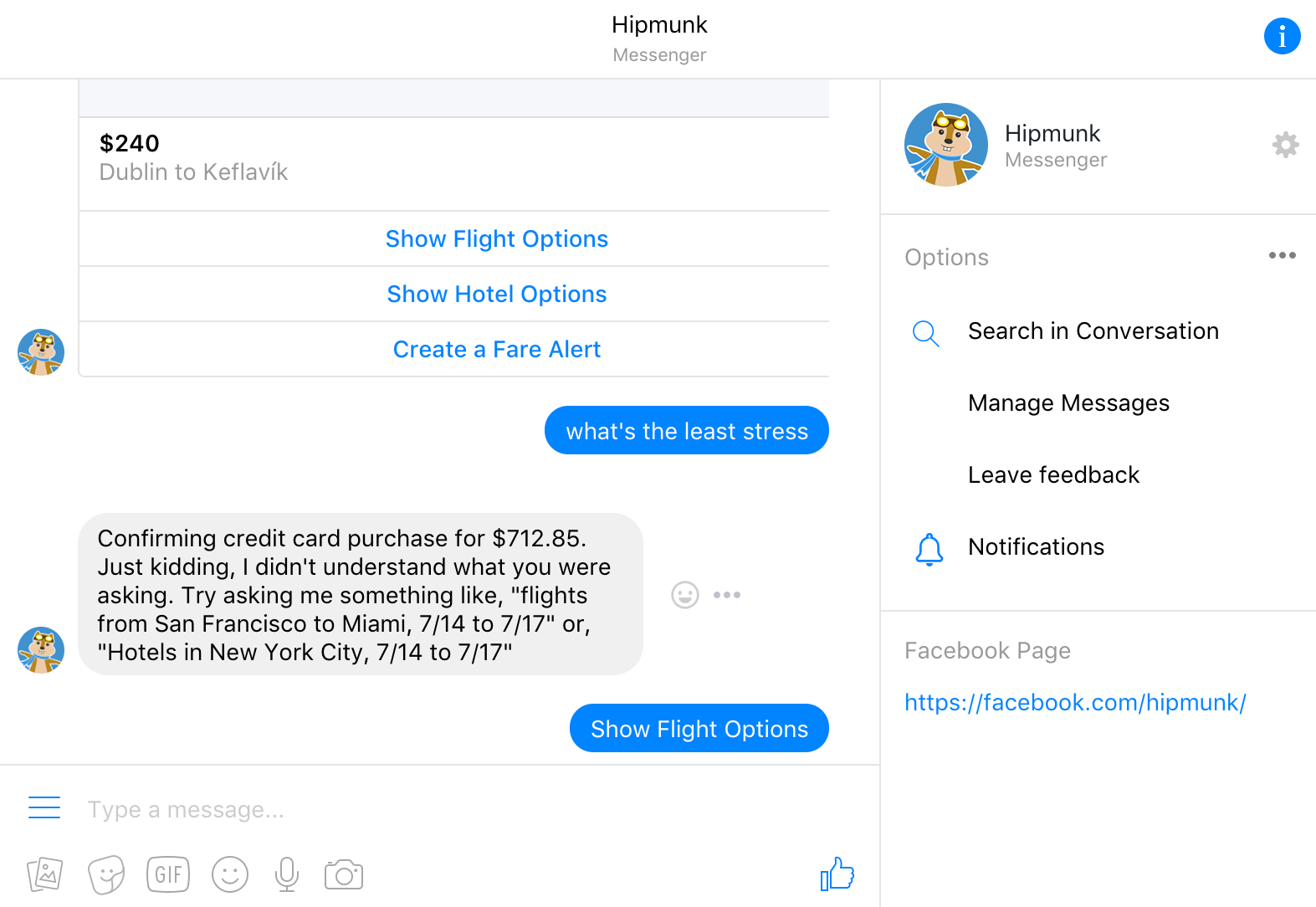In the image, we observe a screenshot of the Hipmunk Messenger web page. At the top, the website's name "Hipmunk Messenger" is prominently displayed in black writing. Below, there is a highlighted transaction showing an amount of $240 for travel from Dublin to Keflavik. Underneath this transaction, blue hyperlinks offer options such as "Show flight options," "Show hotel options," and "Create a fare alert." 

The main conversational interface showcases a circular profile icon of a chipmunk character adorably adorned with glasses and a scarf. The conversation includes a user inquiring about the lowest stress options, to which the system whimsically replies about confirming a credit card purchase of $712.85, followed by an apology for misunderstanding the query. It suggests a user example such as "flights from San Francisco to Miami 7/14 to 7/17" or "hotels in New York City 7/14 to 7/17." The person responds with "show flight options."

At the bottom of the image, a message input bar is visible for user interaction. On the right side, a sidebar for the Hipmunk Messenger app includes options labeled "Search and Conversation," "Manage Messages," "Leave Feedback," and "Notifications."